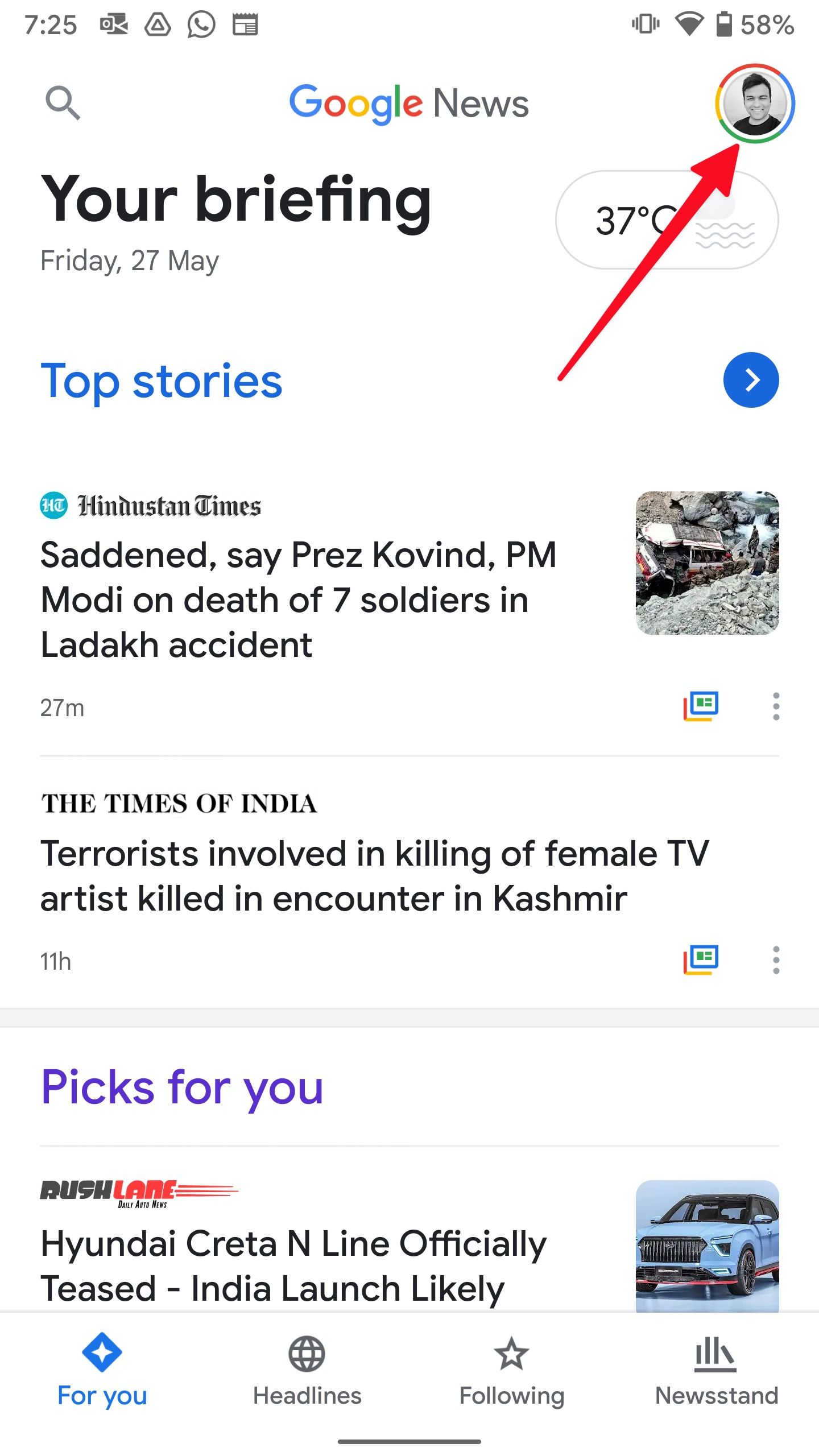A mobile screenshot of the Google News app displays a personalized news briefing. At the top right corner, the user's profile photo, encapsulated in a round circle, is prominently highlighted with a large red arrow, indicating its location. The upper left side of the screenshot features the bold text "Your briefing" followed by the date, "Friday, 27th of May," and the current temperature beside it. Below this header is the "Top stories" section, listing two news stories with an option to view more by clicking on a blue circle with a left-pointing arrow.

Towards the bottom, the "Pics4U" section is highlighted in purple, indicating it has been selected, showing a preview of an article. The bottom of the screenshot features the navigation bar of the app. The "For You" tab is active, highlighted in blue, positioned to the left of other sections: "Headlines," "Following," and "Newsstand," which are all in gray.